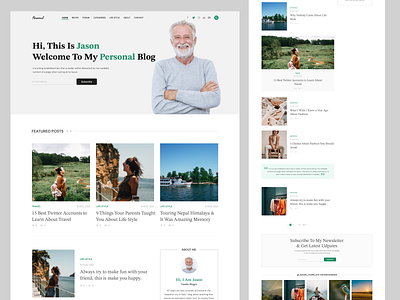A screenshot of a blog website displays a Caucasian man in his 50s or 60s with a welcoming message: "Hi, this is Jason. Welcome to my personal blog." The top of the page features a navigation menu with unreadable options due to the image's small size. Underneath Jason's greeting, the blog's header highlights "Featured Posts," accompanied by various images of a woman in outdoor settings, such as a meadow and multiple beach locations. On the right side, a sidebar showcases additional photos of the woman in different poses with accompanying text, though the details are too small to discern. This image could either be an actual snapshot of Jason's personal blog or a template sample demonstrating a potential blog layout created by a web development company.